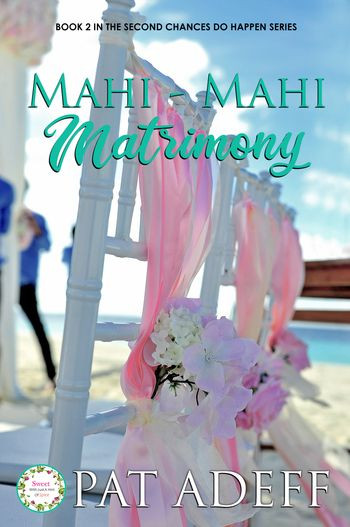This is a highly detailed and vibrant book cover image for "Mahi Mahi Matrimony," the second book in the "Second Chances Do Happen" series. The cover features a close-up photograph of two ornate white chairs, decorated elegantly with pink and white silk ribbons and bouquet arrangements of pink and white flowers near the seats. The chairs are set on a light sandy beach under a clear blue sky, with the ocean visible in the distance, indicating a beach wedding setting. The background showcases a sunny day with some blurred people on the left side of the image, dressed in black pants and blue shirts, adding to the lively atmosphere. 

At the top of the image, in small black text, it reads, "Book 2 in the Second Chances Do Happen series," followed by the title "Mahi Mahi Matrimony" in large, teal, creative fonts, with the word "Matrimony" written in cursive, also in teal. At the bottom left corner, there is a small white circle adorned with floral designs, though the text inside is too small to read clearly. To the right of this logo, at the bottom of the image, the author's name, Pat Adiffe, is displayed prominently in large white capital letters. The overall design is bright, pastel, and summery, perfectly capturing the joyous and romantic essence of a beach wedding.